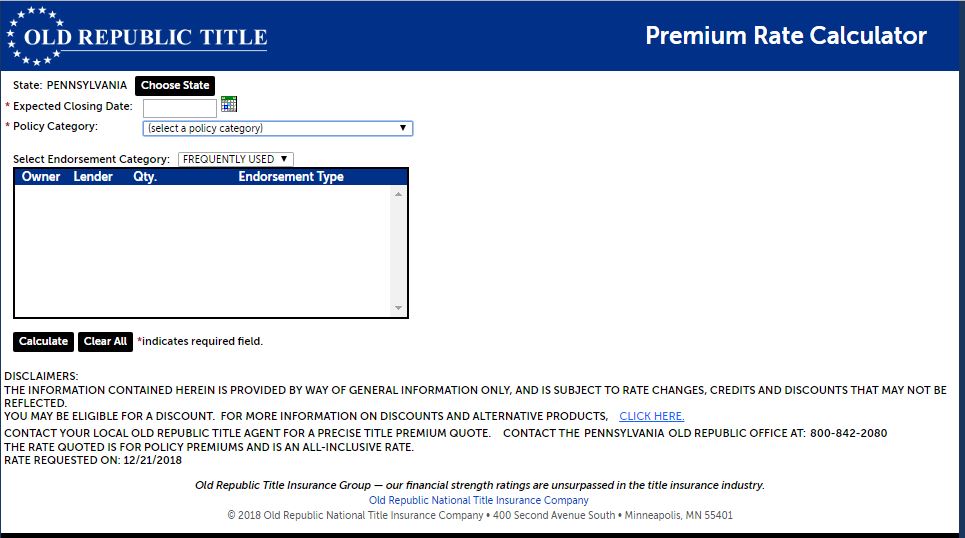This image features a webpage from the Old Republic Title Company, showcasing a premium rate calculator designed for loan estimates. The page has a blue header bar with the Old Republic Title Company logo on the left and the text "Premium Rate Calculator" in white on the right. Below the header, the form prompts the user to select their state and expected closing date for the loan, which could be related to a mortgage. 

Next, there is a dropdown menu for selecting the policy category, followed by an option to choose an endorsement category that allows for frequently used lenders. At the bottom of the form, there are buttons to calculate the rate or clear all inputs. Additionally, a disclaimer at the bottom of the page notes that the rates are subject to changes, credits, and discounts which may not be reflected in the calculator's results. Overall, this tool provides users with a general estimate of potential premium rates for loans involving a title, such as a car purchase or mortgage.